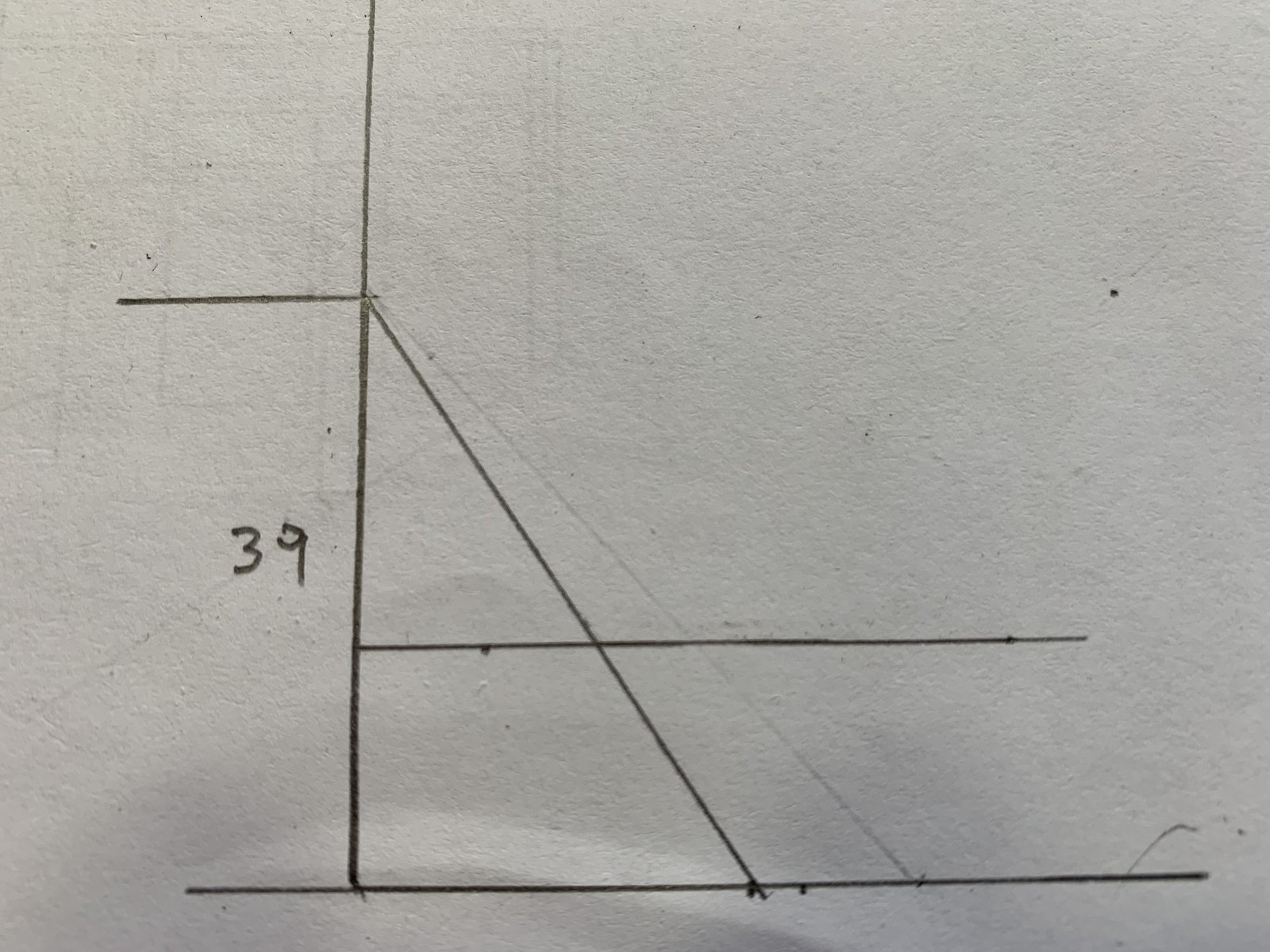A plain white piece of paper serves as the canvas for a pencil sketch, characterized by multiple erasures and redrawn lines. The image features a number "39" prominently displayed, suggesting it could be part of a mathematical exercise or diagram. The left side of the paper is dominated by a large line intersected diagonally, creating a triangular shape above and a slanted square below. Additionally, two disconnected lines on the left side contribute no clear form to the overall composition, further adding to the abstract, somewhat incomplete appearance.